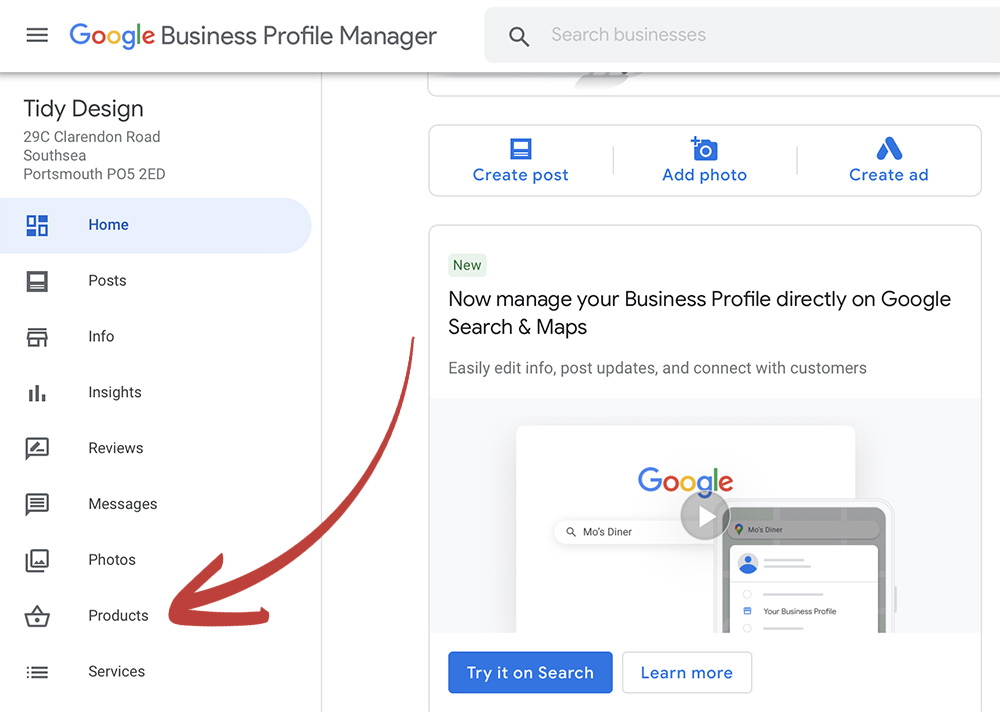The screenshot captures the interface of the Google Business Profile Manager website. At the top of the page is a white banner featuring a hamburger menu icon (three horizontal lines stacked) on the left, followed by the "Google" logo in its signature primary colors. To its right, the banner reads "Business Profile Manager" in clear, black text.

Adjacent to this title is a search bar labeled "Search Businesses," accompanied by a magnifying glass icon. Directly beneath the search bar is a thin horizontal line.

In the left sidebar, "Tidy Design" is prominently displayed in bold text, with "29C Clarendon Road," "South C Portsmouth," and the postal code "PO5 2ED" listed beneath it. The sidebar also includes a navigation menu with the following options: Home (highlighted in blue), Post, Info, Insights, Reviews, Messages, Photos, Products, and Services. A red arrow points specifically to the "Products" option.

The main section of the website greets users with the options to "Create Post," "Add Photo," and "Create Ad," all presented in blue text. Below this, a green banner with the word "New" introduces a new feature: "Now manage your business profile directly on Google Search and Maps. Easily edit info, post updates, and connect with customers." At the bottom of this section, blue and white banners guide users towards more information with "Learn More" links.